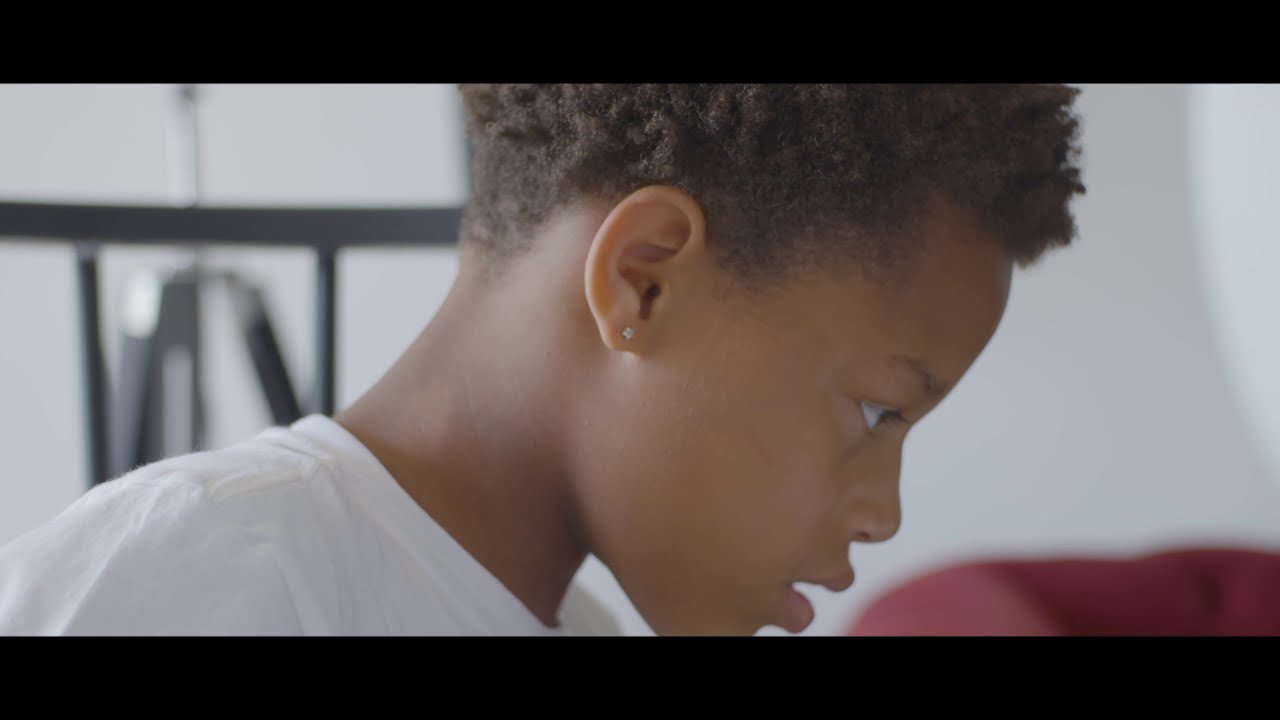In the image, there is a young African-American boy with smooth dark brown skin and short curly coiled brown hair. He is facing to the right with his mouth slightly open and appears to be staring intently at something in the bottom right corner. He is wearing a small diamond stud earring in his right ear and a white t-shirt. The background features a white wall with a distinctive black railing behind his head, consisting of a curved horizontal piece with two straight black posts below it, between which is some sort of device with diagonal components. To his right, out of focus, is a piece of red furniture, likely a couch. The image is letterboxed with black borders at the top and bottom, giving it a cinematic feel.